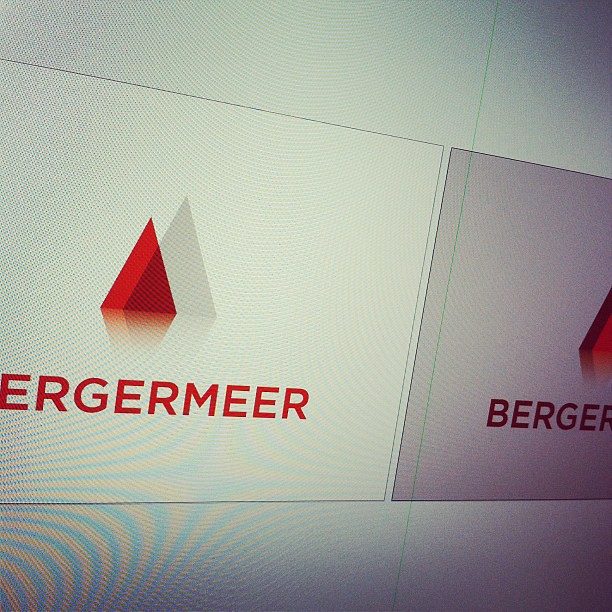The image depicts a mostly white and grey background featuring bold, red text that reads "Bershmer" prominently displayed. Above this word, there is a red triangle pointing upwards, accompanied by its shadow which is slightly larger and aligned to the side. The image appears somewhat blurry or distorted, indicating it was likely captured from a screen or monitor. Despite the slight blur, the image remains bright and clear enough to discern its contents. There are no additional numbers, words, or shapes present in the overall setting.